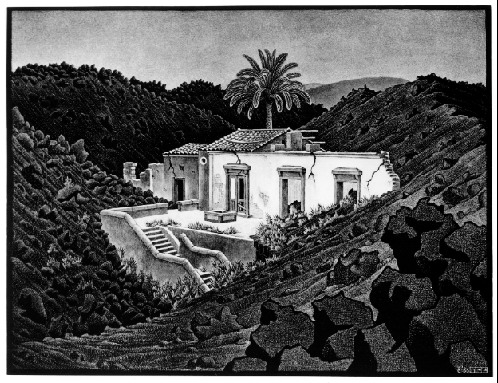This black and white painting, possibly a finely detailed sketch made using tiny dots, depicts a white, stone house nestled amidst steep, crisscrossing hills that are black and green. The house, appearing slightly in ruins, has several entryways and an outdoor stairway leading to an upper courtyard. It has a tile roof that is partially missing on the right-hand side, revealing cracks in the walls and foundation. A towering coconut, or perhaps king palm tree, stands behind the house, adding a touch of southern European flair. The hillsides, adorned with indistinct gray trees and shrubbery, frame the house. The sky above is a light green hue. The painting's border is black, with a thin vertical black pinstripe running along the right-hand side and an unreadable print or watermark in the lower right-hand corner.